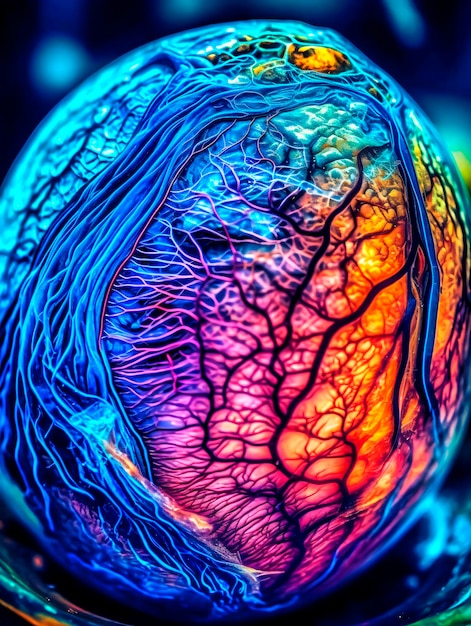The image depicts a stunning computer-generated scene, showcasing a large egg-shaped structure with neon colors and intricate vein-like patterns running throughout. The veins are vividly colored in varying shades of dark and light blue, purple, pink, teal, turquoise, magenta, green, yellow, and orange. The interior of the egg appears to be softly glowing with radiant red and pink hues, enhancing its ethereal appearance. The veins, reminiscent of capillary networks or tree branches, are intricately woven across the surface, creating a mesmerizing and dynamic web of neon light. This captivating image evokes a fantastical vision, possibly of a dragon's egg, and suggests that under a black light, its colors would vibrantly glow, further emphasizing its surreal and otherworldly beauty.